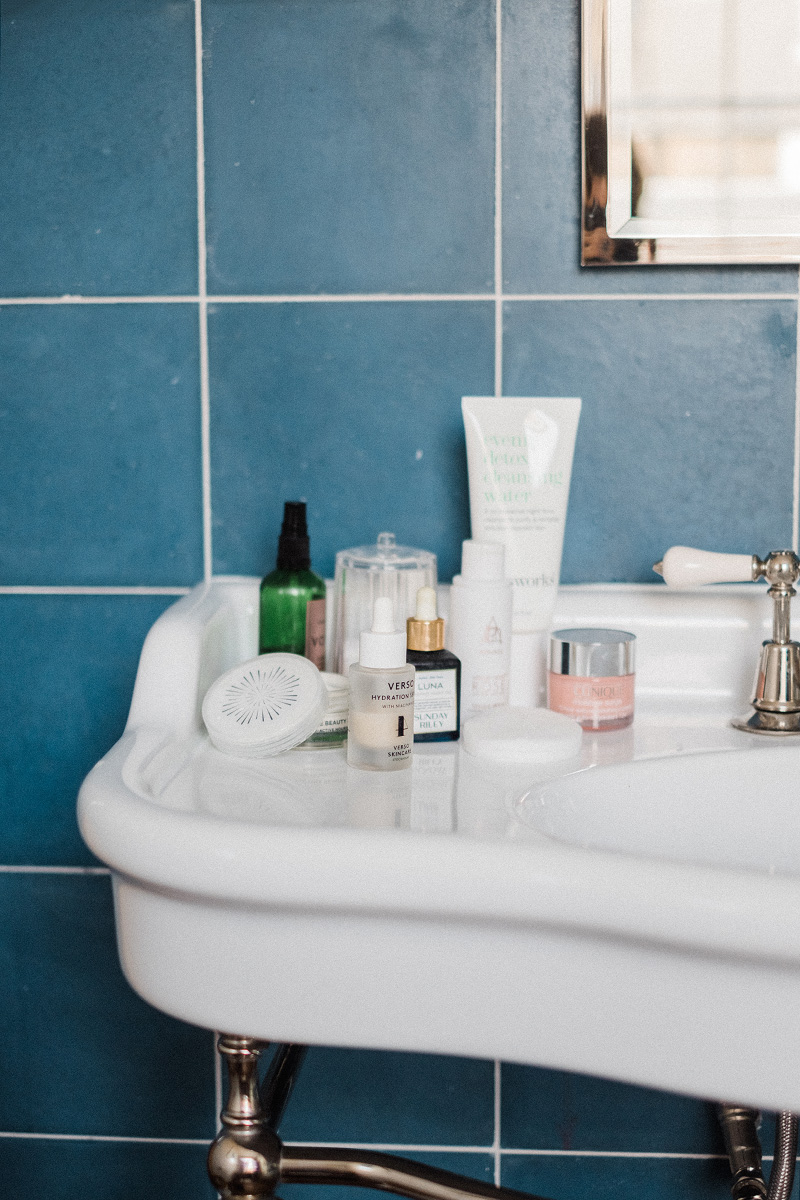A close-up photograph captures one half of a white porcelain bathroom sink, accentuated with decorative silver-toned metal legs. The medium blue tiled wall behind the sink adds a vibrant background, partially reflecting a person with brown hair in the mirror situated in the upper right corner. The circular sink, though partially visible, seamlessly integrates into a compact countertop featuring a subtle ridge designed to prevent water overflow. Adorning the left side of the small counter are an assortment of toiletries: a green spray bottle, a stand-up lotion tube, a small pot with a pink substance protected by a silver cap, two smaller spray bottles, a circular sponge, and another round object. A sleek silver-toned faucet with a white ceramic handle completes the basin's elegant yet functional design.